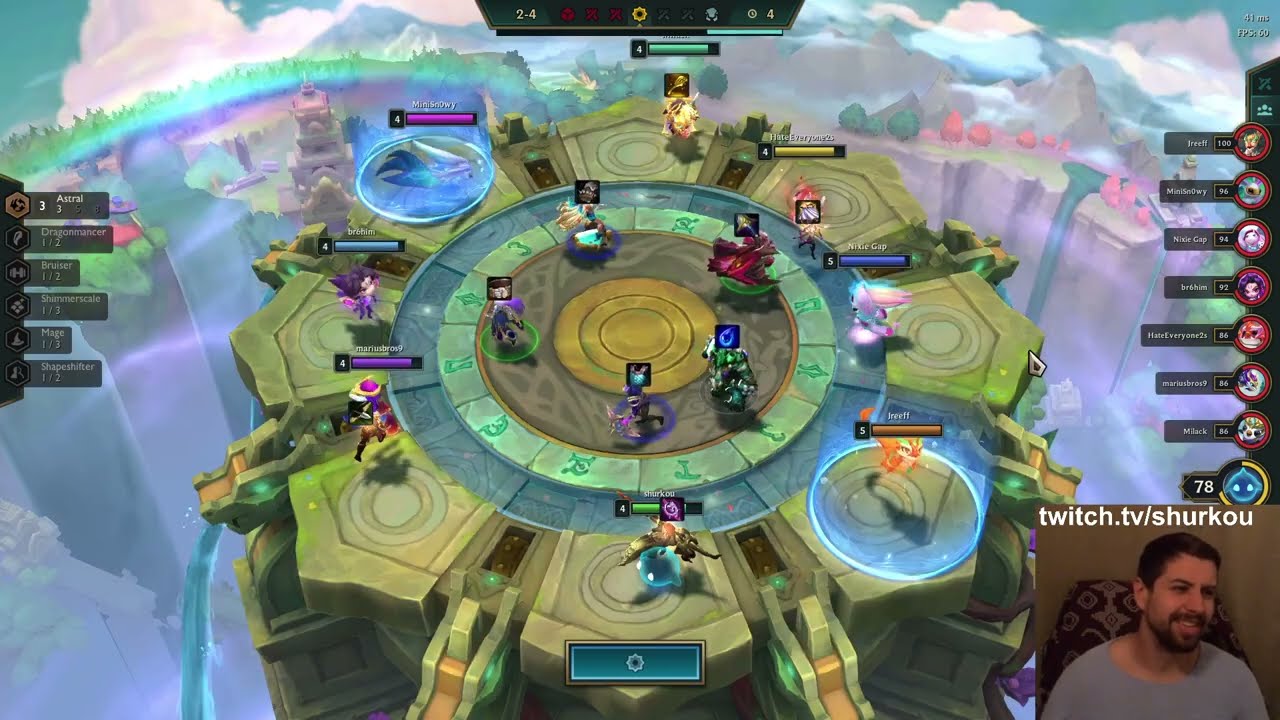This detailed caption combines elements and shared details from all three voice descriptions, focusing on the most repeatedly mentioned aspects:

"A wide rectangular image of a video game screen showcases a dynamic scene set against an aerial view of a mountainous, metallic landscape adorned with scattered clouds. Dominating the center is a large, circular, flower-like structure with multiple concentric rings of varying colors—gold at the center, transitioning to gray, teal, light blue, and green. Each ring features several player characters, indicated by square emblems, foreign language symbols, or horizontal bars in colors such as yellow, blue, purple, turquoise, lavender, and green. Plenty of information is displayed on both sides of the image; the left side stacks player levels, including one labeled '3' at the top, while the right side features characters aligned vertically along with names and circular icons.

In the bottom right corner, a smaller square inset shows a live streamer with dark hair and a beard, dressed in a gray shirt, slightly tilting his head to the right, seated in a red and gray chair. Above this inset, white letters spell out 'twitch.tv/shurkou,' slightly above the number '78' beside a light blue sphere adorned with two blue dots and a semicircle of gold. The overall interface also includes menu bars and various interactive buttons, creating an intricate and engaging gaming scene."